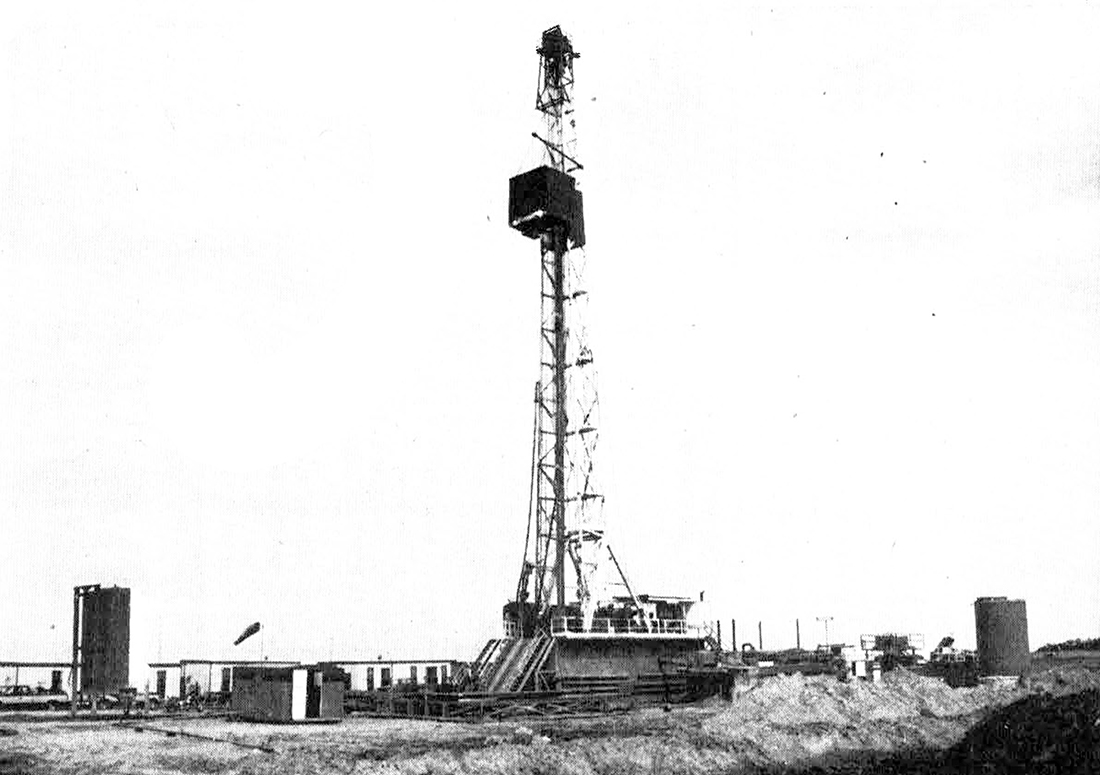The black-and-white photo, possibly vintage, depicts an outdoor scene dominated by an industrial structure, likely an antenna or an oil rig, marked by its stark contrast and graininess. The centerpiece of the image is a tall, metal tower extending upward into a clear, white sky. At the top of the tower, there appears to be a small box-like platform. The ground surrounding the tower is flat, composed of grass and dirt patches, indicative of an open field setting. To the left of the tower, a small shed with a white door is visible, and further in the background, there are silos and trucks, suggesting an industrial or oil field environment. Additionally, an orange flag, commonly used to signal low-flying aircraft, is seen fluttering above the site. The sky is featureless, adding to the photo's starkness, and the overall scene gives a sense of an expansive, somewhat barren landscape with a few scattered industrial elements.